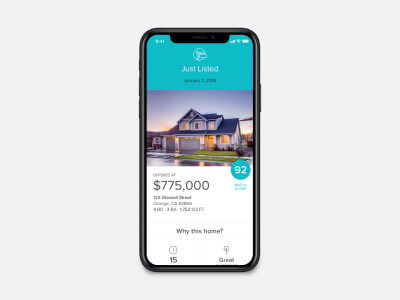This image is a detailed mock-up for a real estate mobile app, presumably used by or representing a real estate company or an app-building service. The backdrop of the mock-up is a neutral gray, which helps to highlight the main subject: a smartphone showcasing the real estate app interface. 

The top section of the app screen is designed with a blue header featuring the real estate agent's name prominently at the center. Just below the agent's name, small black text provides additional information, though the details are not entirely clear. 

Centrally positioned on the screen is an image of a property, giving users a visual focus and hinting at the primary function of the app—property listings. 

In the lower-left corner of the screen, the property rating is displayed, likely to offer users immediate insight into the property's quality or desirability. Adjacent to this, towards the bottom left, are the property's price and additional details, making key information readily accessible. 

Finally, centered at the very bottom in small black letters, is the call-to-action text “Buy this home,” clearly indicating the app's purpose and utility as a platform for facilitating real estate transactions. This well-structured layout highlights the potential of the app as a valuable tool for both real estate professionals and clients.